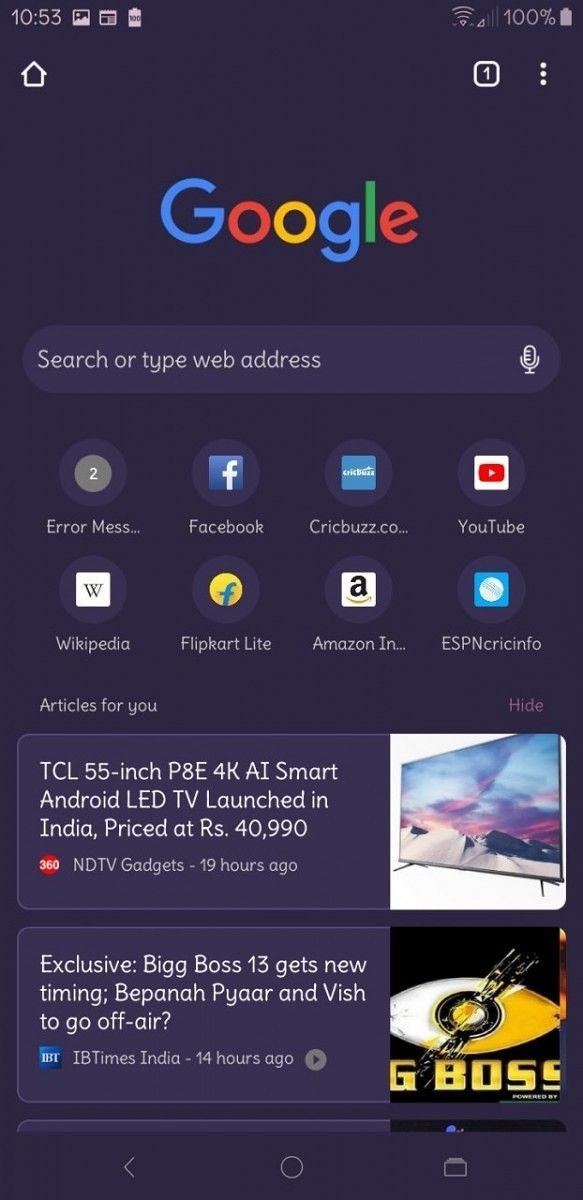A detailed screenshot taken at 10:53 AM on an Android device captures the Google search homepage. In the background, the photo app remains open. The device has a full battery charge at 100%, Wi-Fi is enabled, and there is a cellular connection with only one bar of signal strength. The search tab is active but empty, indicative of no current queries. Frequently visited sites and bookmarks are visible, featuring icons and links to Facebook, CrickBuzz.com, YouTube, Wikipedia, Flipkart, Amazon, ESPN Cricinfo, and an error message page.

Additionally, recommendations for "Articles for You" are displayed, including headlines from NDTV Gadgets and IB Times India. Noteworthy articles include an NDTV Gadgets post about the launch of the TCL 55-inch P8E 4K AI Smart Android LED TV in India, priced at Rs 40,990, from 19 hours prior, and an IB Times India article about exclusive changes to Bigg Boss 13's timing and the conclusion of 'Vapana PR in Vish,' posted 14 hours ago. The Android navigation buttons (Back, Home, Overview) are also visible at the bottom of the screen.